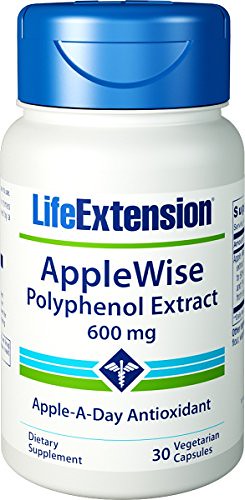The image displays a supplement bottle designed to promote health and wellness. The bottle is predominantly white with a contrasting blue cap, providing a sleek, clean appearance. The label, primarily white with blue and green accents, prominently features the brand name "Life Extension" at the top. Below the brand name, the product is identified as "AppleWise Polyphenol Extract, 600 mg." Further down, the label highlights the supplement's benefits with the phrase "Apple-A-Day Antioxidant." The lower section of the label indicates that the bottle contains "30 Vegetarian Capsules" and denotes it as a "Dietary Supplement" in smaller font.